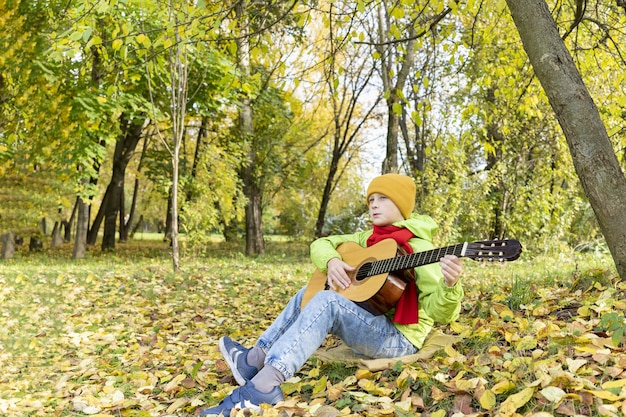In the photograph, a young boy, approximately 10 to 13 years old, is seated on a small pillow or bag beneath a diagonally positioned tree in a serene, natural setting. His bright attire includes blue jeans, blue sneakers with white stripes, gray socks, a green sweatshirt with a hood, a knotted red scarf, and a mustard-yellow beanie. He holds a classic wood-style guitar, possibly playing it, while looking pensively into the distance. The ground is carpeted with fallen leaves in varying shades of yellow, brown, and green, indicating the early stages of autumn. Surrounding him are numerous trees with sagging branches adorned with yellowish-green leaves, and in the background, a meadow is visible through the foliage, adding to the peaceful and pastoral ambiance of the scene.